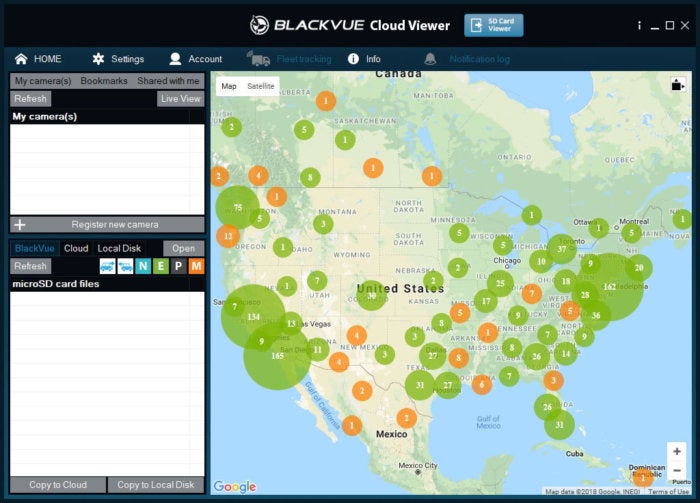The image depicts an interface for the "BlackVue Cloud Finder," prominently displayed at the top with a black banner and white text. Adjacent to this title is a blue button featuring an icon of a door and an arrow, labeled "5D Card Viewer." Below, a blue navigation bar includes options such as Home, Settings, Account, Fleet Tracking, Info, and Notification Log.

On the left side, there's a section titled "My Cameras," featuring a blank space reserved for camera registrations, marked by the text "Register New Camera."

The centerpiece, dominating the right side of the interface, is a detailed map of North America, including the United States, Canada, and Mexico. This map is punctuated by numerous green and orange circles, each containing numbers, indicating specific points of interest or activity. The most significant clusters of these circles are found around New York, California, Washington (Seattle), and Denver, Colorado. The circles are predominantly situated along the outer regions of the United States, with fewer clusters spread across Canada and three notable points in Mexico. The specific meaning of these circles remains unclear, but their distribution suggests a focus on certain high-activity areas.